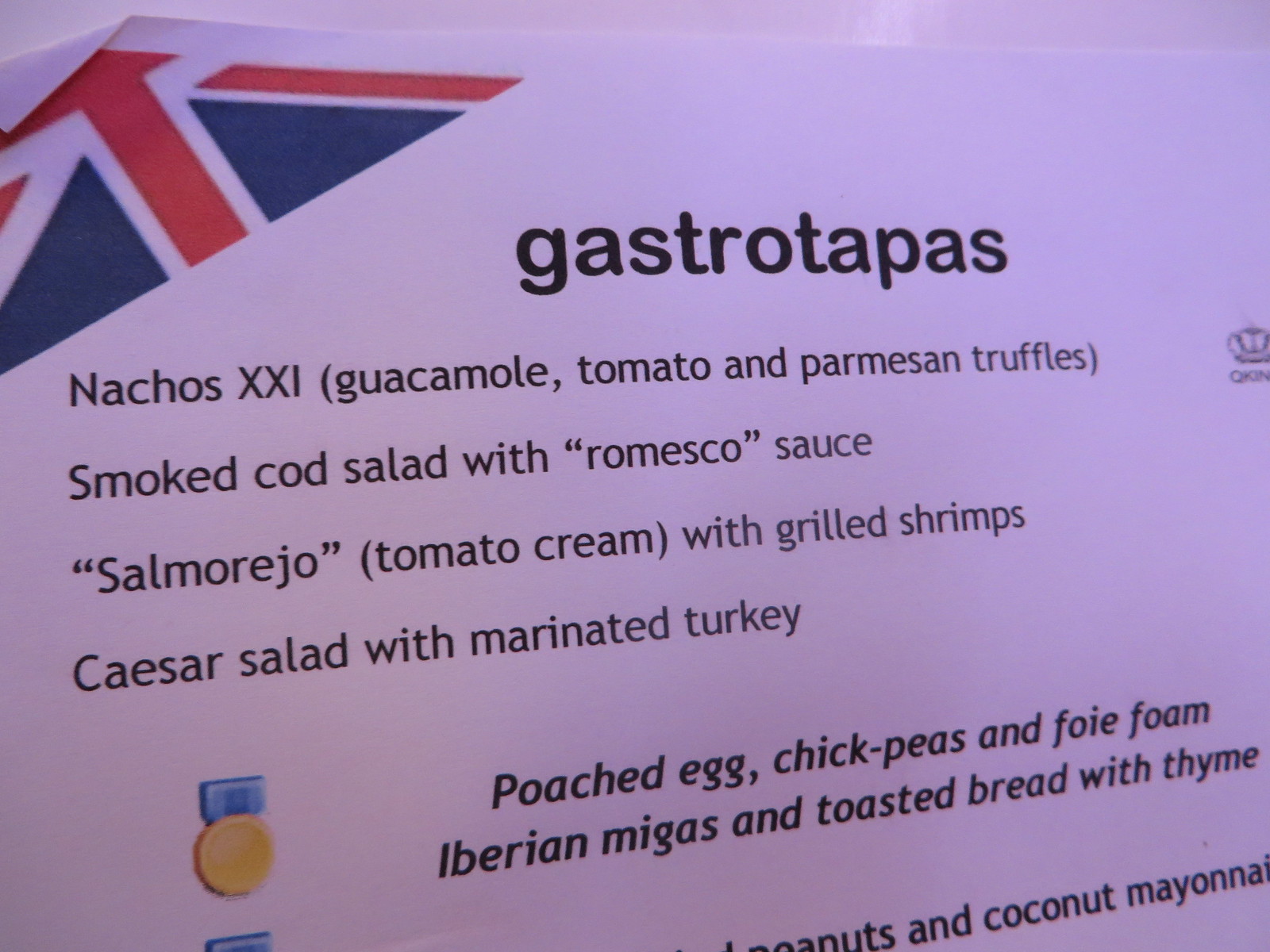This wide rectangular photograph showcases a portion of a paper menu against an off-white background. The menu’s edge is visible only at the top, slightly folding at the top left corner where a partial image of a British flag is displayed, featuring a blue background with a red cross and red X. At the top of the menu, in bold lowercase letters, it reads "gastro tapas." Below, in sequence, are menu items: "nachos XXL" with guacamole, tomato, and parmesan truffles; "smoked cod salad with romesco sauce;" "salmorejo" - a tomato cream with grilled shrimps; and "Caesar salad with marinated turkey." Toward the bottom, in a bolder font, are additional items: "poached egg, chickpeas, foie foam," "Iberian migas," and "toasted bread with thyme." An image of a gold medal is also present underneath the text.